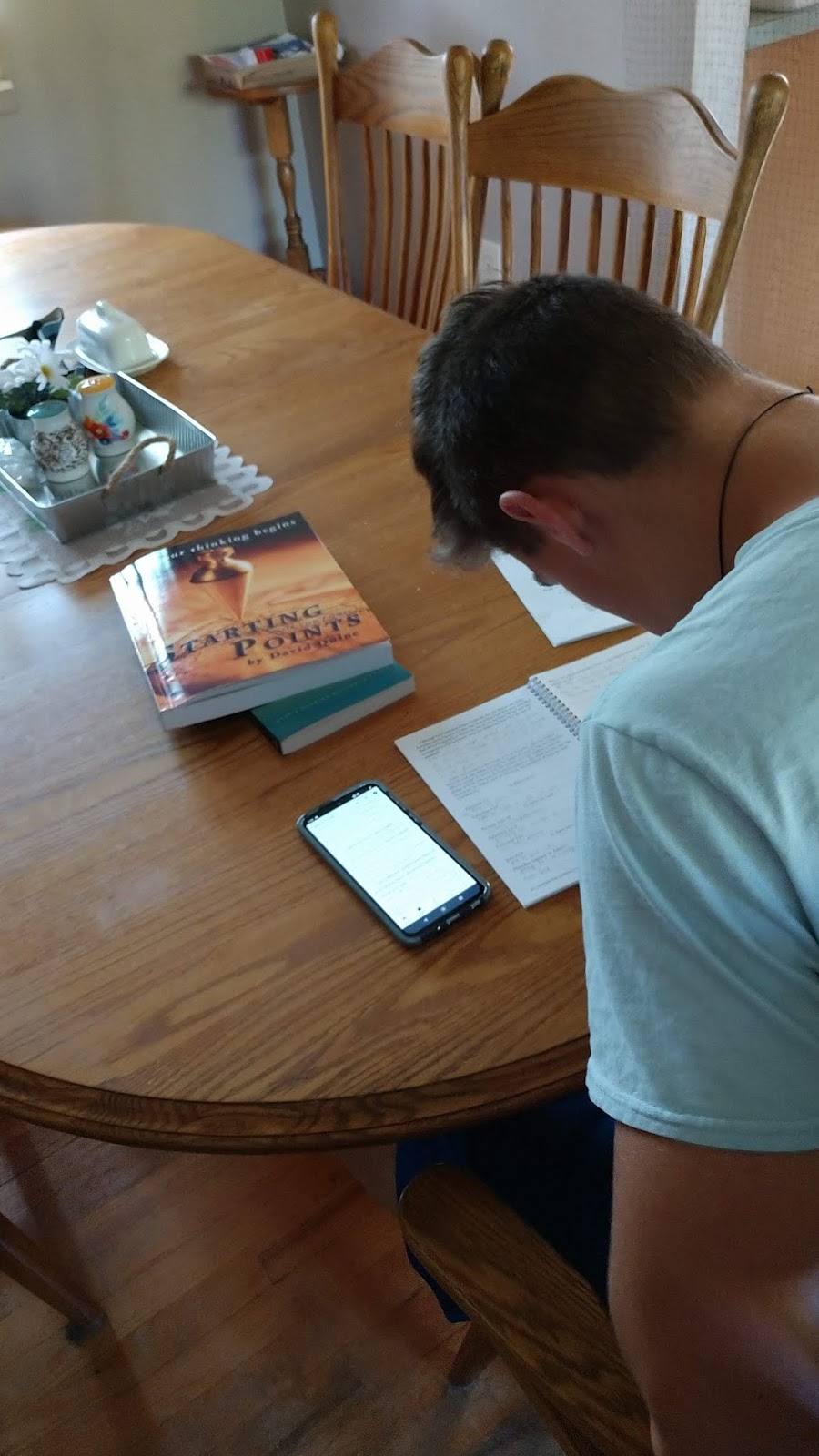An over-the-shoulder photograph captures an individual diligently working at a golden-hued, oval-shaped wooden dining table. The table, affixed with a honey-glow finish, features a platter of assorted knick-knacks, including white ceramic salt and pepper shakers with blue and yellow lids, flowers, and other small items, all neatly arranged on a white, squared doily. Visible beyond the top right of the table is an adjacent floor area through an open doorway. Two matching wooden chairs with solid backs and vertical railings are partially visible at the top of the frame. The focal point of the image is a book titled "Starting Points" that lies in front of the man, who is engrossed in his open journal filled with printed questions. His phone, screen lit, sits nearby, possibly serving as a secondary reference tool for his note-taking session.